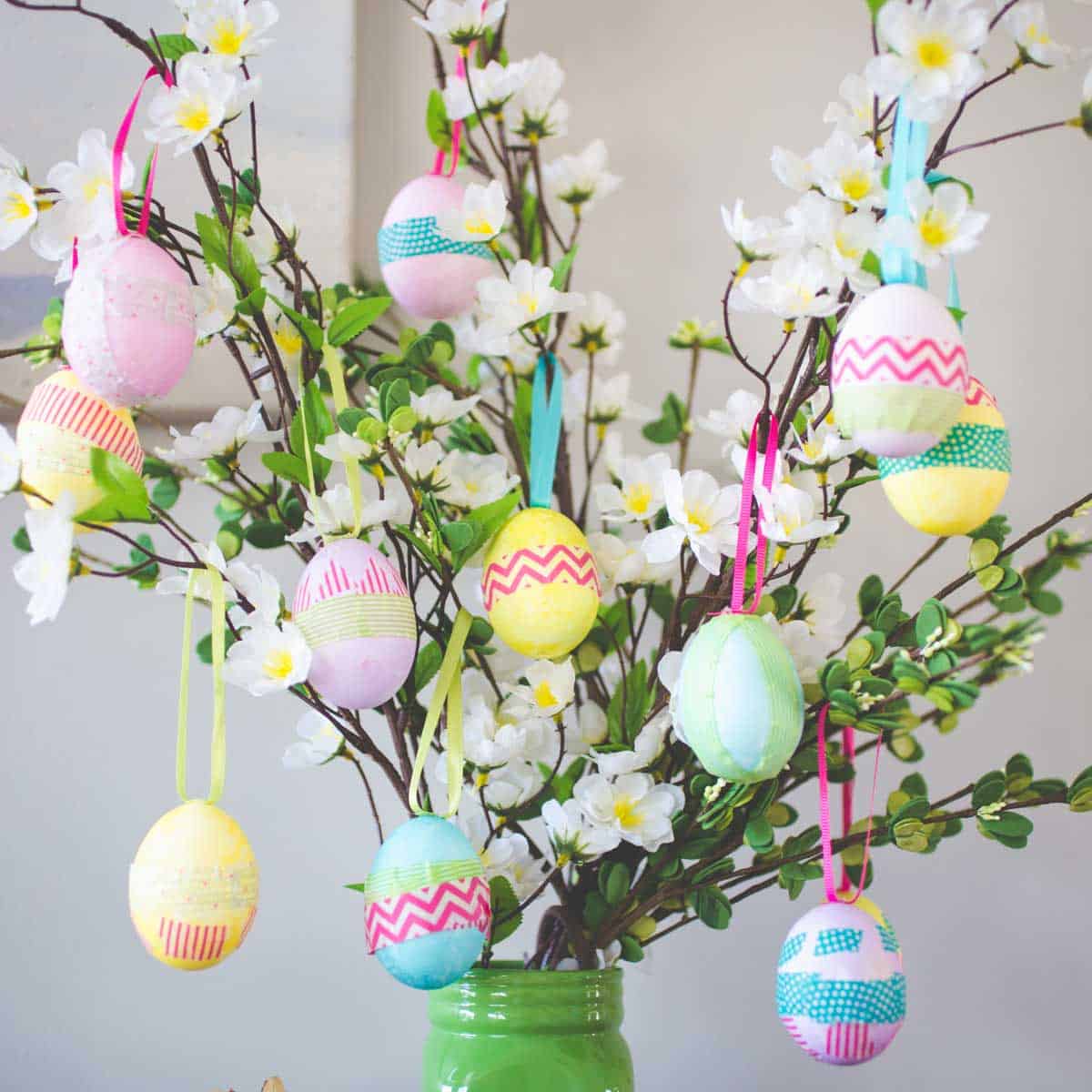In this image, a green mason jar anchors the composition, set against a gray background. Emerging from the jar are numerous fake branches, including some designed to resemble boxwood with green leaves. Interspersed among these are other branches adorned with white flowers that have yellow centers. Adding an Easter theme, the branches are festooned with about ten colorful, decorated plastic Easter eggs. Each egg, adorned with stripes and dots, hangs delicately from ribbons in a variety of pastel hues including pink, blue, yellow, and green, enhancing the festive and decorative aesthetic of the arrangement.